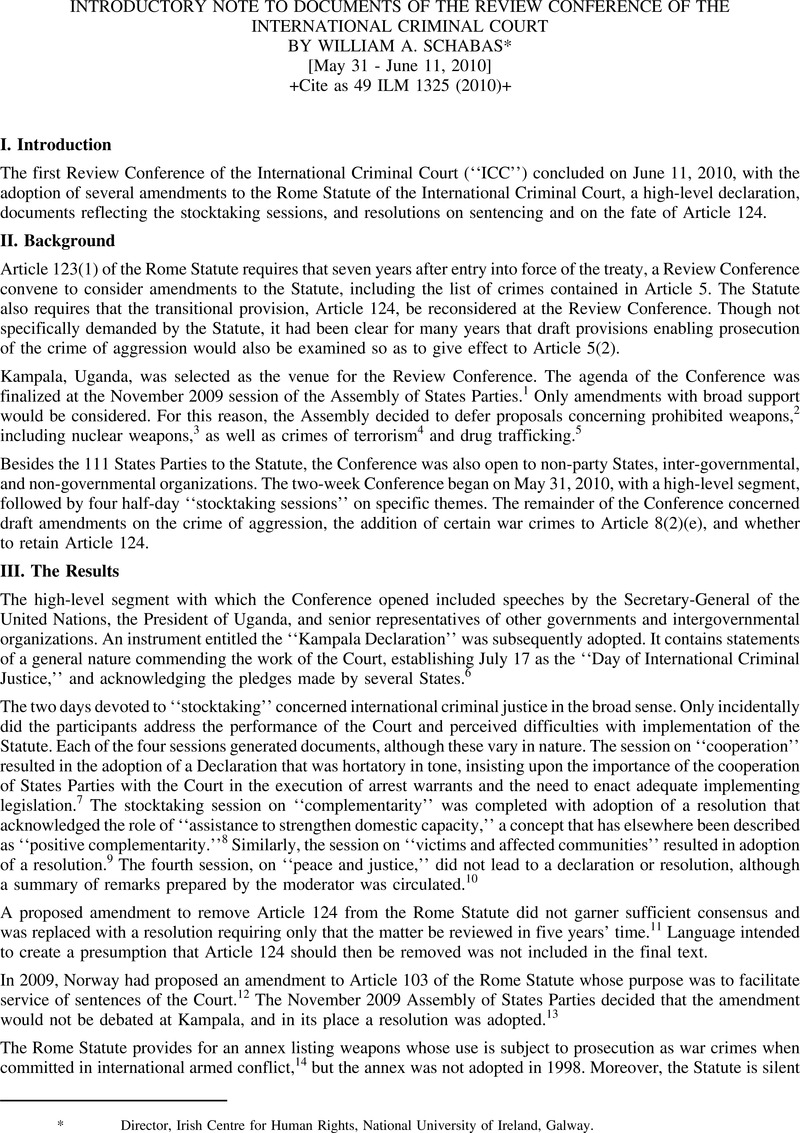The image is a scanned criminal document, presenting black text on a white background. It is titled "Introductory Note to Documents of the Review Conference of the International Criminal Court" by William A. Schabas, dated from May 31 to June 11, 2010. The document begins with an introductory section, briefly summarizing the proceedings of the First Review Conference of the International Criminal Court (ICC), which concluded with the adoption of several amendments to the Rome Statute. These amendments are encapsulated in a high-level declaration document that reflects the stocktaking sessions and resolutions on sentencing and on the fate of Article 124.

Following the introduction is a detailed background section, explaining that Article 123 of the Rome Statute mandates a review conference seven years after the treaty's entry into force to consider amendments, including adding new crimes under Article 5. It notes that Article 124's transitional provisions were also up for reconsideration and discusses the long-anticipated examination of draft provisions enabling the prosecution of the crime of aggression related to Article 5. The document mentions Kampala, Uganda, as the chosen venue for the review conference, with the agenda finalized during the November 2009 session of the Assembly of State Parties. Only amendments with broad support, excluding those concerning prohibited weapons, terrorism, and drug trafficking, were to be considered.

The final included section, titled "Results," is the most extensive, comprising five paragraphs. It elaborates on the outcomes and implications of the conference resolutions. The text additionally references a citation, "CITES 49 ILM 1325, 2010," which appears near the document's top.